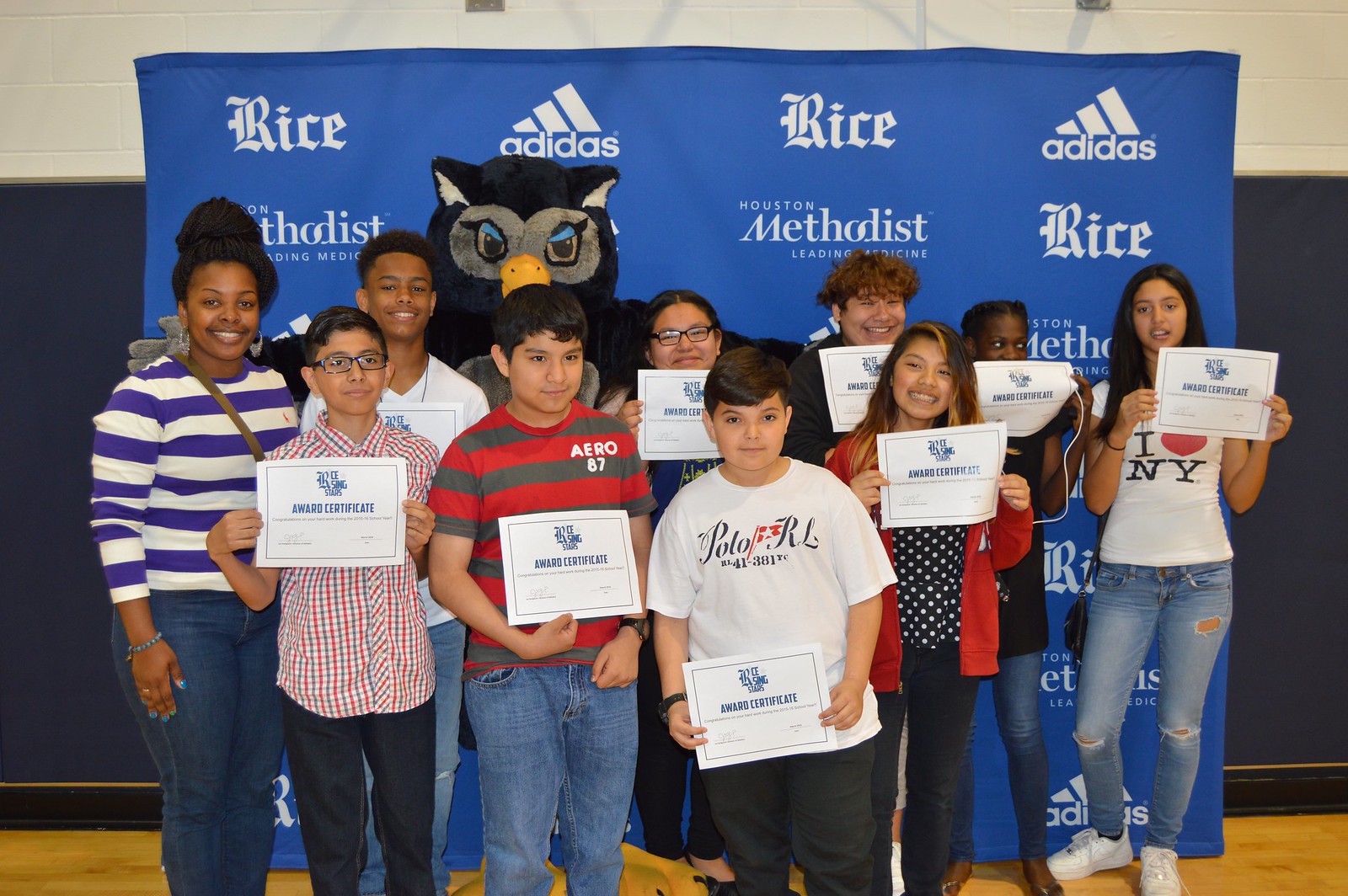A group of 11 children, comprising six boys and five girls, are standing on the wooden floor of a school gymnasium, receiving awards. They are all holding white sheets representing their certificates, smiling proudly at the camera. Behind them, a dark blue banner adorned with white text from various sponsors, including Rice, Adidas, and Houston Methodist, hangs prominently. The banner features repeated rows of the sponsors' names. Central to the backdrop is the school's owl mascot, adding a touch of school spirit. The children are dressed in diverse outfits, with some notable attire including a child in an "I Love New York" shirt and another in an "Arrow 87" striped shirt. To the left stands a teacher dressed in a white and blue striped shirt, and two other adults are positioned at the back. The scene captures a celebratory moment in what appears to be a gymnasium set up for an awards ceremony.